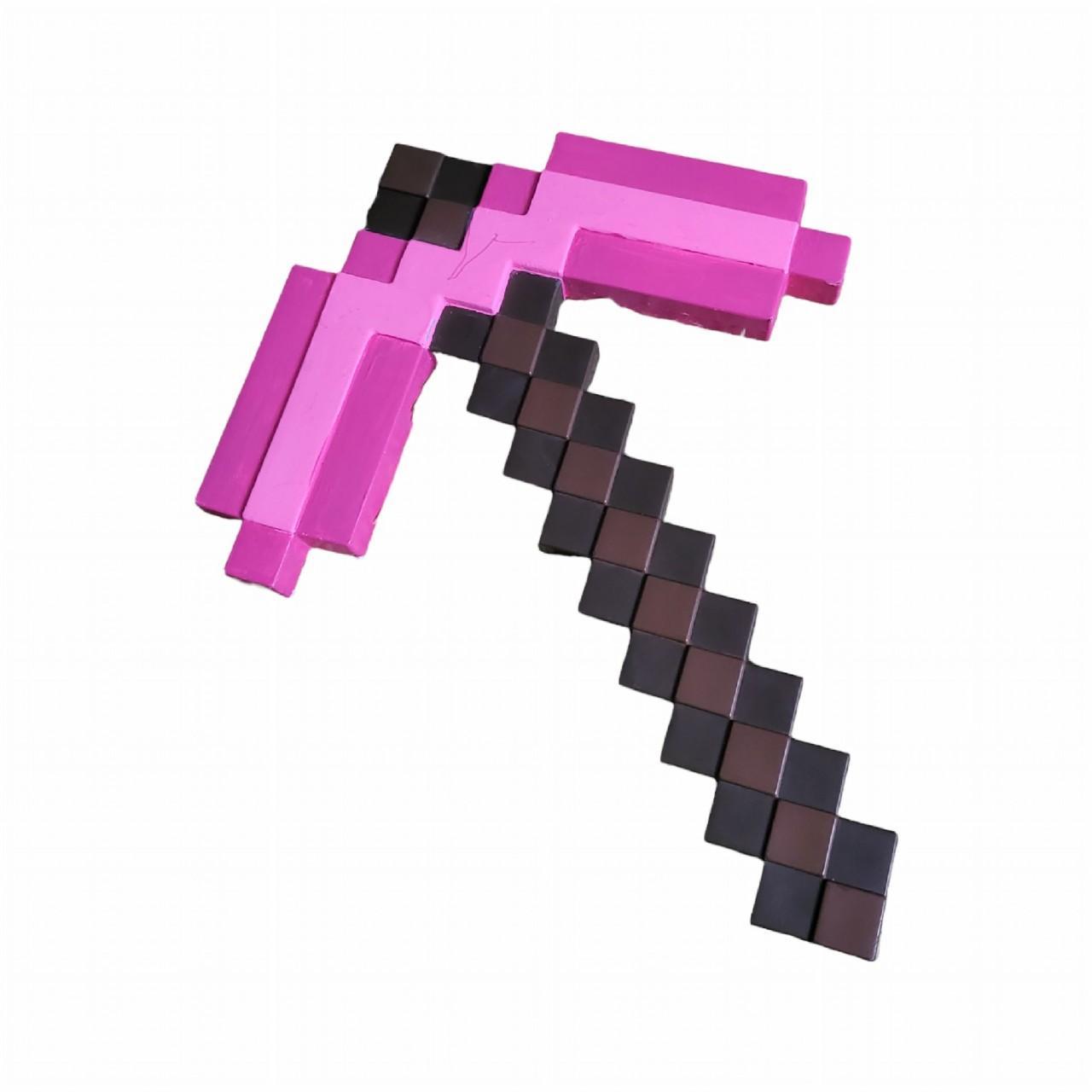The image features a handmade Minecraft-themed pickaxe crafted from small cubes, set against a plain white background. The handle is composed of alternating dark brown and light brown squares, creating a checkered pattern that extends the length of the pickaxe. The head of the pickaxe is constructed from a combination of dark pink and lighter pink cubes, arranged to form the distinct pickaxe shape with the axe blade leaning slightly to the upper left. The edges of the pickaxe appear slightly rough and uneven, suggesting some imperfections or possible wear. This detailed, cuboid design evokes the iconic pixelated aesthetic of Minecraft, presenting a visually striking and well-crafted representation of the in-game tool.